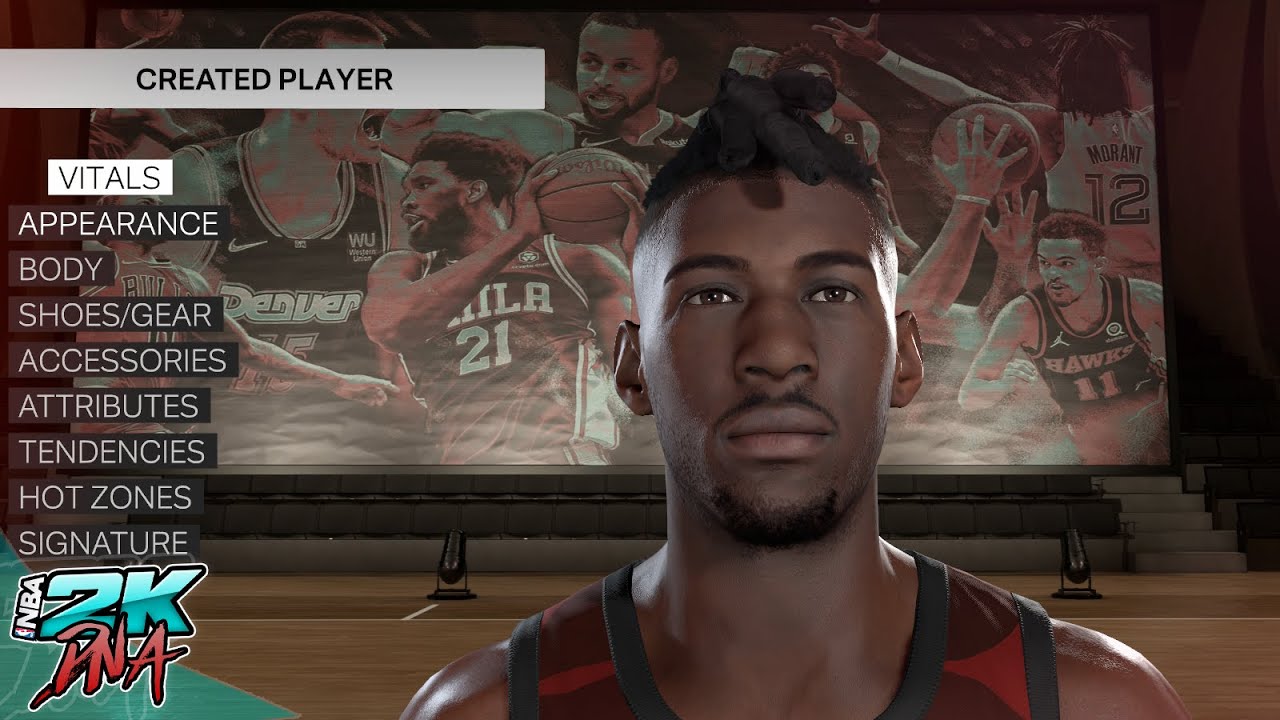Here's a cleaned-up and detailed caption for the image described:

---

This image depicts a customizable player interface from the NBA 2K video game. Displayed prominently in front of a large television screen, which showcases a dynamic collage of various NBA players, the created player stands at the center of the interface. This feature allows users to meticulously design their own basketball player with chosen skill sets. The interface sidebar lists various customization options, beginning with 'Vitals' highlighted in white.

The first section, 'Appearance,' enables users to alter the player’s face, hair, and other physical features. The 'Body' section likely adjusts parameters such as height and weight. Further customization includes 'Shoes' and 'Gears' for selecting the player's footwear and other equipment, as well as 'Accessories' for adding finishing touches.

For gameplay enhancement, the interface includes 'Attributes,' which define the player’s skills, 'Tendencies,' which guide their in-game decisions, and 'Hot Zones,' which indicate areas of the court where the player excels. Additionally, there's a 'Signature' section, possibly allowing users to create unique moves or even personalize a signature move for their player. This elaborate setup signifies the extensive customization options available to gamers, emphasizing the effort involved in crafting a unique and enhanced basketball player.